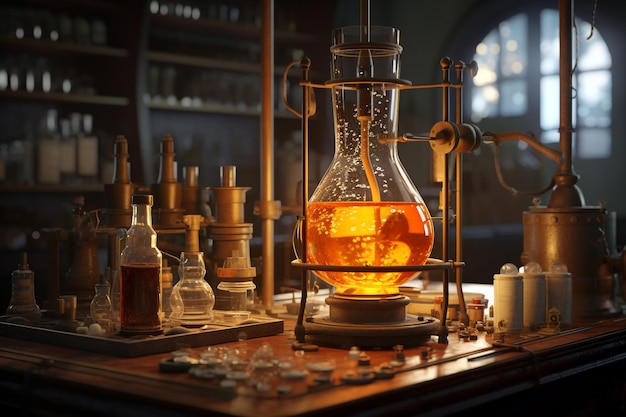This computer-generated image depicts a detailed scene inside a science laboratory, primarily showcasing a chemistry setup. At the center of the image, a large flask, partially filled with a bubbling orange-yellow liquid, is securely held by a metal frame. The liquid appears to be glowing, casting a warm light onto the surrounding area of the desk. Additional chemistry equipment and various smaller containers are scattered around the primary flask, contributing to the authentic lab atmosphere. To the left, shelves lined with numerous glass bottles can be seen, though they are slightly blurred, focusing attention on the central chemistry equipment. On the right side, a double-arched window lets in daylight, though the outdoor view remains indistinct. The overall color palette includes silvers, whites, browns, and yellows, enhancing the scientific environment. The image lacks any visible text, reinforcing the focus on the meticulously arranged laboratory setting.